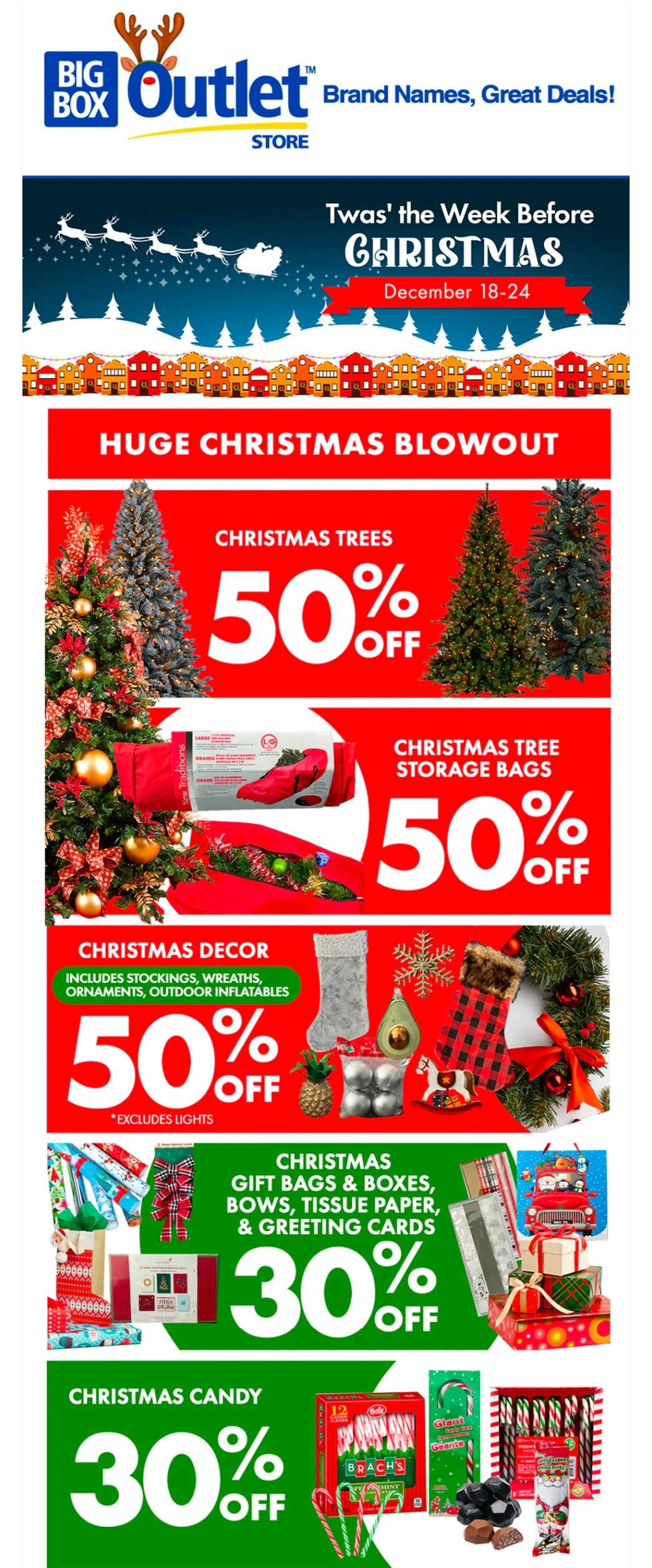The caption has been cleaned up and rephrased as follows:

"A collection of coupons featuring various Christmas-themed advertisements for the Big Box Outlet Store, prominently displayed at the top with a reindeer logo that includes a red nose, two ears, and antlers. Beneath the logo, a yellow swoosh separates 'Big Box Outlet' from 'Store.' The headline reads 'Brown Names, Great Deals!' 

The first callout, set against a picturesque backdrop of Santa and his reindeer flying over a city with pine trees and undulating hills, states, "'Twas the week before Christmas, December 18th - 24th." Below this, the text announces a 'Huge Christmas Blowout' followed by detailed offers:

1. Christmas trees: 50% off 
2. Christmas tree storage bags: 50% off 
3. Christmas decor (including stockings, wreaths, ornaments, and outdoor inflatables): 50% off 

Images of Christmas trees, storage bags, stockings, wreaths, ornaments, inflatables, and various toys complement the offers. 

The next two coupons, set against green backgrounds, advertise:
4. Christmas gift bags, boxes, bows, tissue paper, and greeting cards: 30% off
5. Christmas candy: 30% off, with visuals of candy canes and assorted boxes of candy."